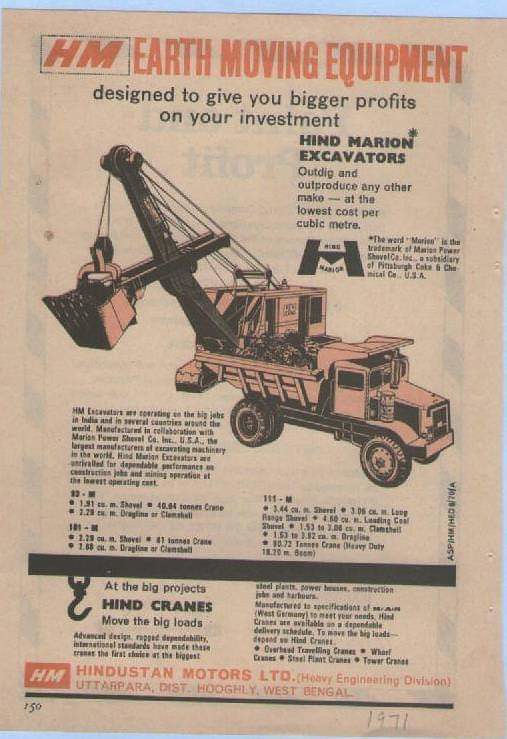This detailed image is a vintage-style advertisement taken from a magazine, specifically page 150 as noted in the lower left corner. The ad, presented in portrait orientation, is for HM Earth Moving Equipment and features bold red text at the top with the letters "HM" italicized and inset into a black rectangle outlined box. The primary headline reads "HM Earth Moving Equipment," followed by a tagline promising bigger profits on investment: "Designed to Give You Bigger Profits on Your Investment."

The centerpiece of the page is a line art drawing of a commercial tractor, intricately detailed with a crane fixed to its chassis, angled to the top left, and equipped with a scoop. This image is printed with a light pink tint, standing out against the black-and-white background. Below the machinery image are two descriptive paragraphs extolling the efficiency and cost-effectiveness of Hind Marion Excavators, mentioning their superior digging and productivity capabilities at the lowest cost per cubic meter.

The layout is complemented by text at the bottom, reiterating the company name, "Hindustan Motors Limited," accompanied by the HM logo and additional address information. The overall design uses black-and-white illustration accented with spot colors such as red and light pink, enhancing the vintage appeal of this industrial advertisement.